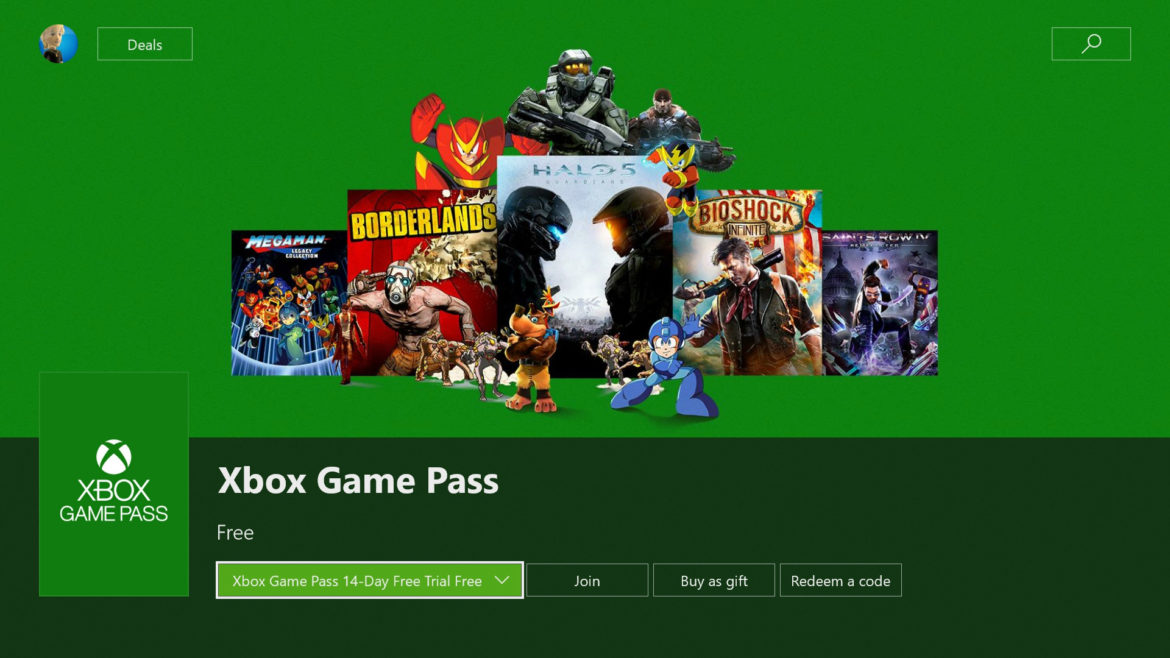This vibrant advertisement for Xbox Game Pass predominantly features hues of green, creating a striking visual appeal. At the top of the image, a circular icon indicates a logged-in user, complemented by a faint white-outlined green box displaying the word "deals" in white text. Positioned on the far right is a conspicuous search box for easy navigation.

The central portion of the image is a lighter shade of green, serving as a backdrop for five prominent game titles. Centered is "Halo 5," a hallmark of the Xbox franchise. To the left are "Borderlands" and "Mega Man," each title evoking its unique gaming legacy. To the right of "Halo 5" are "Bioshock" and another game title that remains indecipherable. Accompanying these titles are character figurines or avatars positioned either above or below the game names, intricately merging with the green background.

On the left side of the image, a green box prominently features the Xbox Game Pass logo and the Xbox symbol, both rendered in clean white. A darker green border frames the bottom of the advertisement, reiterating "Xbox Game Pass" in white text. Below this, it promotes a “14-day free trial,” with options to join, buy as a gift, or redeem a code, making the offering clear and attractive. Through its detailed and visually cohesive design, this advertisement effectively highlights the benefits and notable games available with Xbox Game Pass.